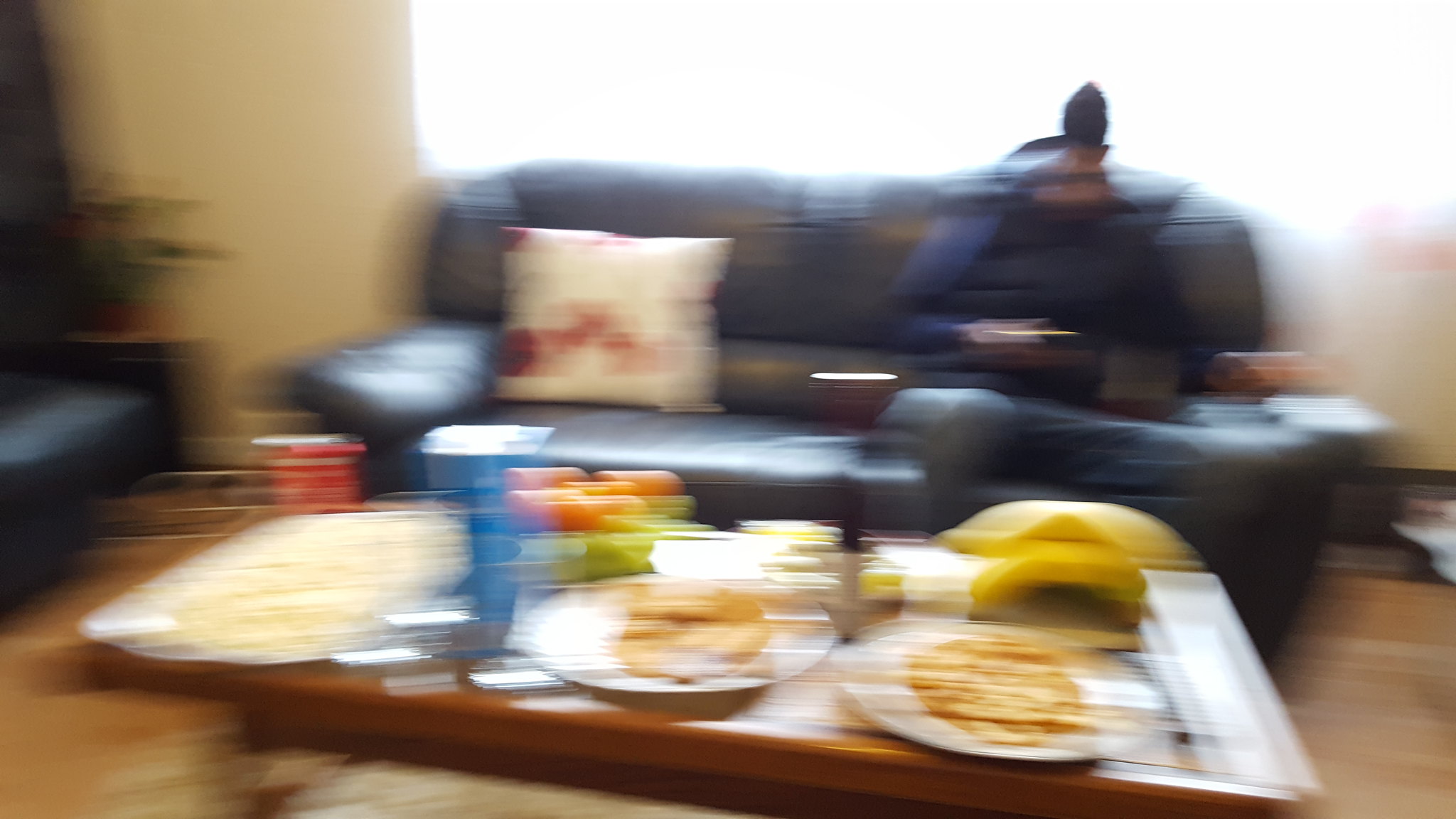In the extremely blurry photograph of a living room, a man wearing a blue long sleeve shirt, black vest, black pants, and a black beanie is seated on the right side of a black leather couch. He is intently looking at his cell phone. On the left side of the couch, a white and red square pillow rests. In front of the couch, there is a low wooden coffee table adorned with plates of food, including what seems to be bananas, crackers, and possibly oranges. A partially visible leather couch is perpendicular to the main couch, extending out of the frame. The floor is pale wood, and the walls are off-white. A bright light streams in from a large window situated behind the sofa. Additionally, there is a green plant against one of the walls, completing the cozy ambiance of the living room.